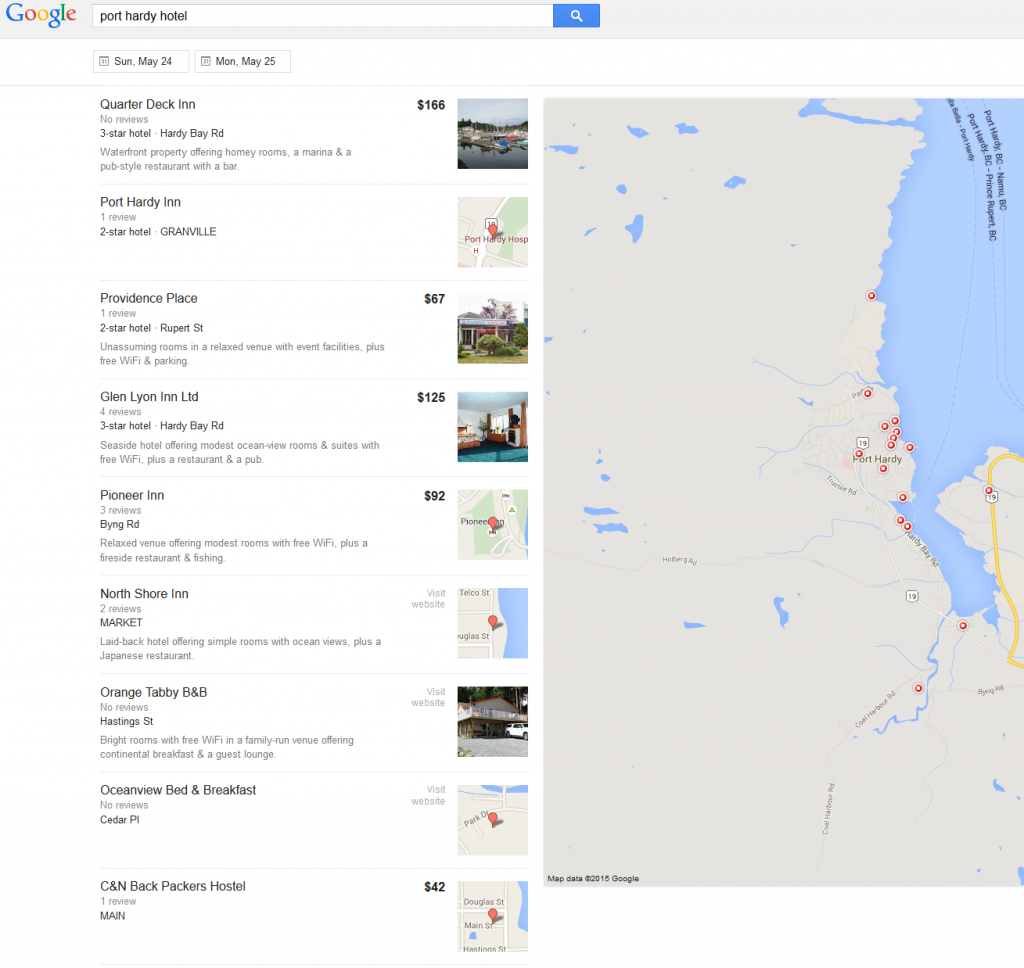The vertically rectangular image displays a Google search page with its screen divided vertically into two sections. At the very top of the image, a narrow gray horizontal banner stretches across, featuring the Google logo in the left corner. Adjacent to the logo is a search field that contains the query "Port Hardy Hotel," followed by the search icon button. Below the search bar, there are two date selection buttons indicating "Sunday, May 24th" and "Monday, May 25th."

Directly beneath the date buttons is a detailed listing of various accommodations in Port Hardy, including:
- Quarter Deck Inn
- Port Hardy Inn
- Providence Place
- Glen Lyon Inn Limited
- Pioneer Inn
- North Shore Inn
- Orange Tabby B&B
- Ocean View Bed and Breakfast
- C&N Backpackers Hostel

On the right side of the image, a full vertical map occupies the entire half, dotted with small red pins representing the locations of the mentioned inns.